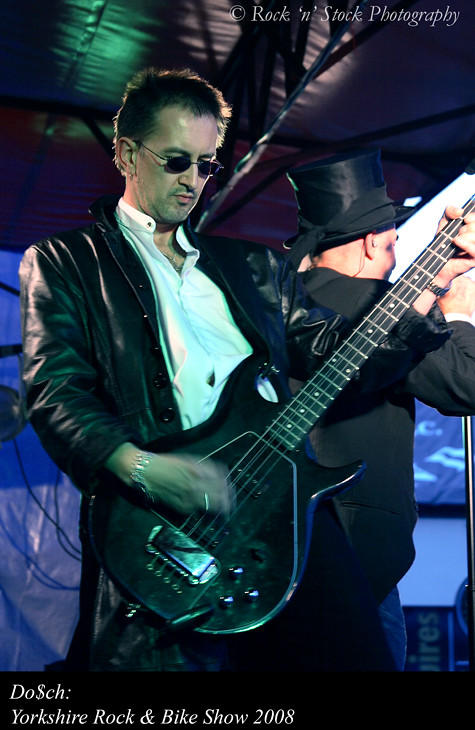This detailed color photograph captures a scene from the Yorkshire Rock and Bike Show in 2008. Dominating the frame is a tall man with short brown hair and black sunglasses, engrossed in playing a black electric guitar. He is dressed in a white open-neck shirt under a black leather jacket, paired with black pants. Adjacent to him, another man stands with his back to the camera, attired in a black jacket and a tall black hat, and wearing blue jeans. The background features a light blue sky, partially framed by a tent-like covering made of black plastic supported by metal trusses. Black electrical cords can be seen in the lower-left corner, hinting at the concert setting. The top of the image is labeled "Rock and Stock Photography," while the bottom prominently displays "D.O. Dallasite, C.H. Cullen, Yorkshire Rock and Bike Show, 2008" in white text.